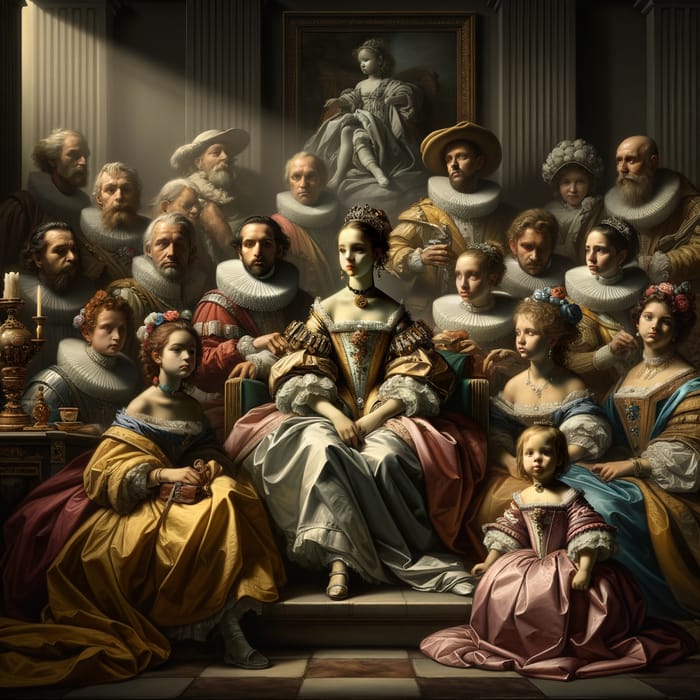This detailed and colorful illustration, possibly computer-generated, presents a royal scene centered around a somber young woman adorned in historical period dress, likely indicating her status as a princess or queen. She sits regally on a chair, looking to the left, and wears a tiara with her hair pinned back. Her attire includes a low-cut, medieval-style gown with flowing pink and cream skirts, puffy sleeves, an embroidered rose on the corset, a black choker with a gold medallion, and dangling earrings. 

Surrounding her are numerous men and women dressed in equally elaborate and luxurious apparel, featuring colors such as pink, white, blue, yellow, gold, red, brown, and gray. The men are seen in frilly lace collars and some with wigs, while many women display hairpieces adorned with flowers and ribbons. Positioned at the left of the young woman is another woman in a flowing yellow gown with a floral crown, who appears to be kneeling or sitting by the central figure's feet. 

In the composition’s bottom right, a small girl in a formal pink dress, similar to the central woman's attire, gazes out directly at the viewer. Additionally, in the very back of this saturated image, an oil painting depicts a young child sitting, adding to the antique and regal atmosphere of the scene. The design, color, and overall setup suggest it might represent an elaborate royal portrait.